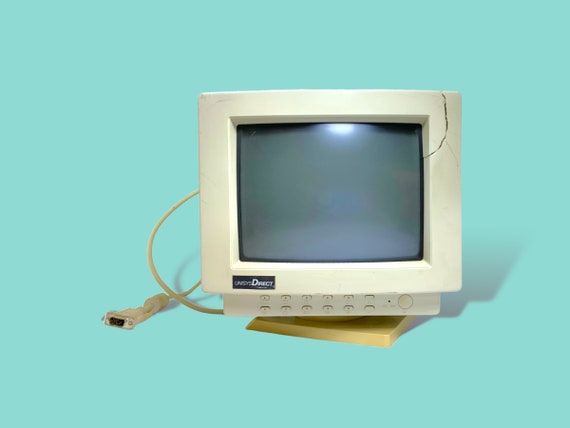The image depicts a very old, almost square computer monitor that dates back to at least the 1990s or earlier. The monitor is characterized by its wide, slightly rectangular off-white plastic frame and features a prominent, approximately four-inch-long crack in the upper right-hand corner, descending towards the cathode ray tube (CRT) screen itself. There's an illegible label in the lower-left corner of the frame and a series of control buttons, possibly six per row, on the bottom of the frame, used for adjusting screen parameters like height and width. The monitor rests on a gold-colored swivel base, which is slightly off-center. On the left side of the monitor, a DB9 computer plug protrudes from the back. The background is a solid sky blue, providing no additional context.